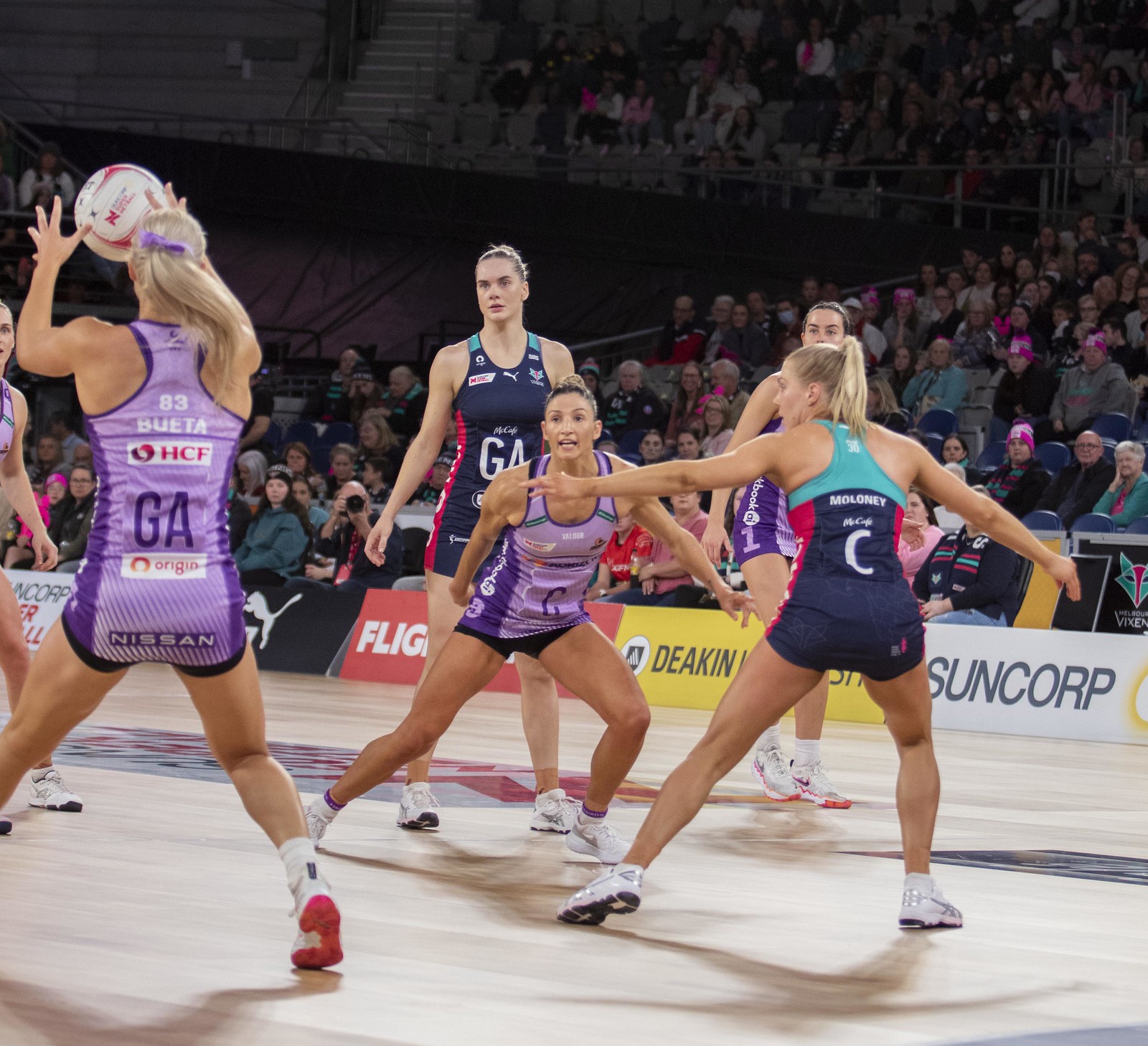The image depicts an indoor sports arena during a professional or semi-professional match involving female athletes. The court features a parquet floor, typical of indoor sports settings, and is bordered with various sponsor advertisements like Flight, Suncorp, and others partially obscured. The scene captures mid-game action with players fully engaged in their sport, which involves a ball and the use of hands, though it’s not clearly volleyball or basketball due to the absence of a net and the unique ball and court setup.

Two teams are distinguishable by their uniforms: one team wears mostly purple outfits with "Nissan" sponsorship and a player with "BUETA" on her back, while the other team is adorned in dark blue with turquoise accents, and the word "Maloney" visible on one uniform. Both teams are positioned on the same side of the court, suggesting a dynamic play scenario. The athletes are clad in very short shorts, white socks, and sport-specific shoes. Surrounding the court, a crowd of spectators can be seen in the stands, engrossed in the unfolding match. A ball is suspended in the air, creating a focal point of the image, just between the hands of a player in purple who appears ready to catch or intercept it.